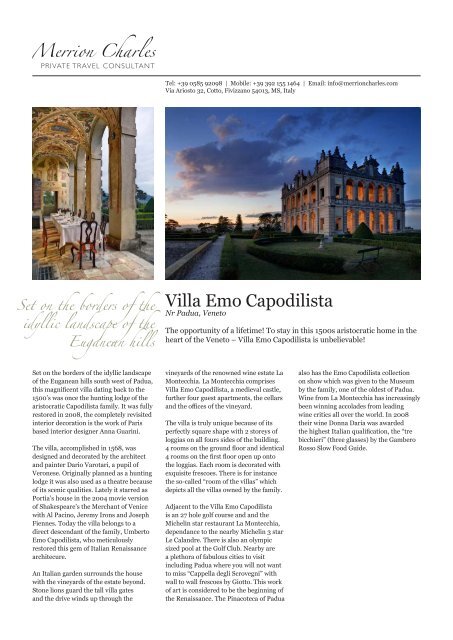This detailed advertisement page from a magazine showcases Villa M.O. Capodilista, a stunning hotel situated in Padua Veneto, Italy. The header at the top left reads "Mary and Charles, Private Travel Consultant," and provides their comprehensive contact information including telephone, mobile, email, and address. The page features two large, captivating images. The first image depicts an elegant dining area inside the villa, adorned with majestic arches and an intricately designed ceiling. The second image captures the villa's breathtaking exterior at sunset, highlighting its illuminated, castle-like structure with a pointed roof, surrounded by green grass and a quaint walkway under a picturesque blue sky with clouds. Below the images, the text describes the villa's prime location "Set on the borders of the idyllic landscape of the Aegean Hills," followed by an in-depth article detailing the lavish features and offerings of Villa M.O. Capodilista.